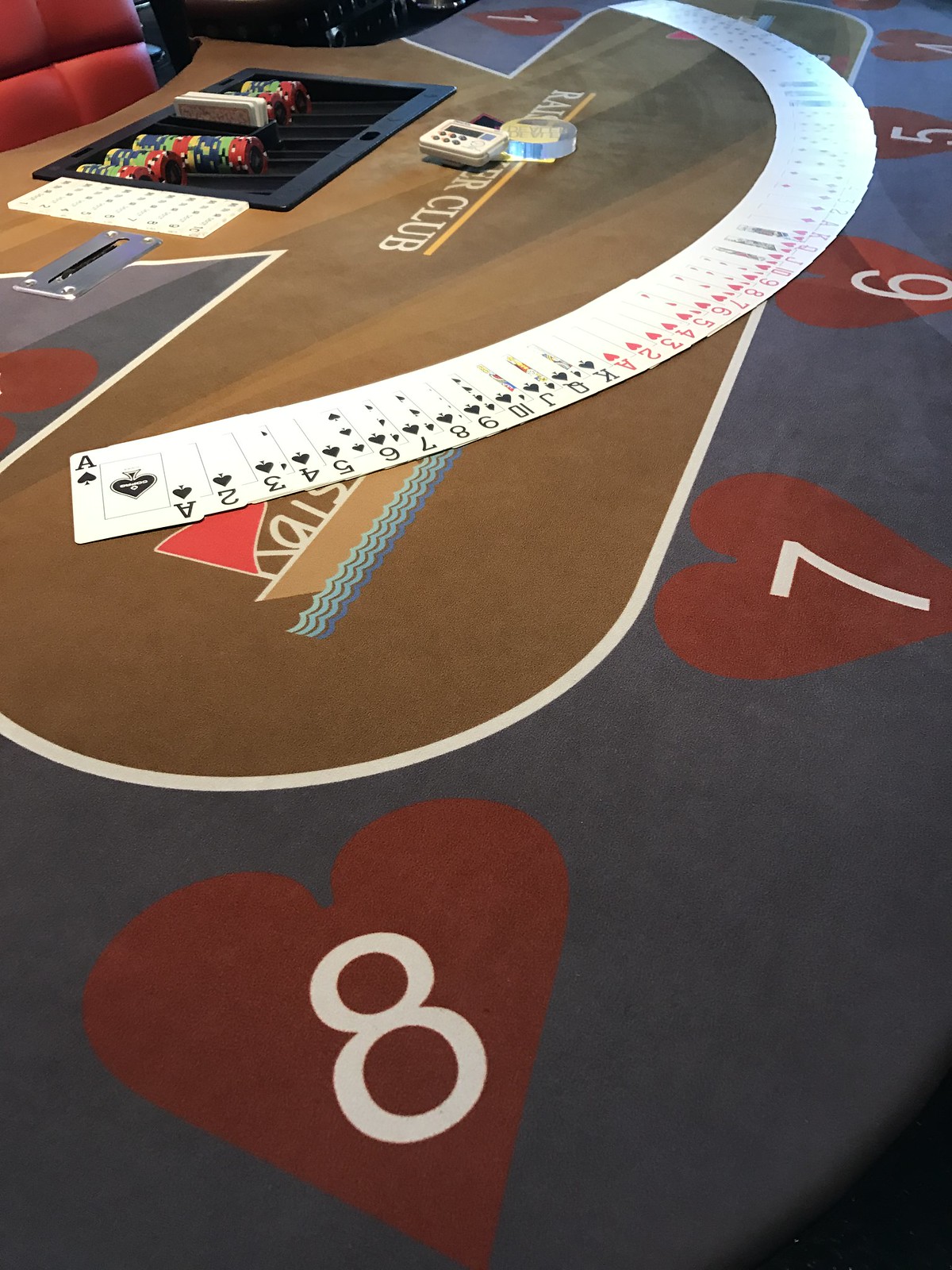This image appears to be taken from a slightly elevated angle, presenting a vertically-oriented, rectangular view. In the background, there's a visible red computer chair, featuring four distinct, plush segments that suggest it is quite comfortable. 

Positioned in front of this chair is a brown desk with a black inset, resembling how a sink is integrated into a countertop. This black section includes a small panel and several items are placed inside, alongside a noticeable white object – possibly hinting at additional functionality. 

The setting is framed by a gray rug or carpet mat highlighted with red hearts around its border. Notably, these hearts contain white numbers counting down from 8 to 4. 

Central to the scene are several gathered items, including a visible sign or plaque that partially reads "Club," though the preceding word is obscured and begins with the letter "R." Additionally, a deck of playing cards is spread out in an overlapping manner, with the numbers of each card clear despite their layered arrangement.